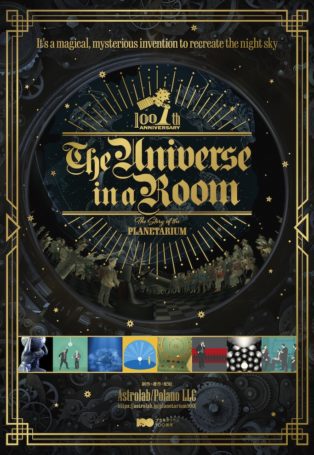This is a portrait-oriented poster with a richly detailed Art Deco-inspired design, mainly using black and charcoal gray tones with gold accents. The poster celebrates the 100th anniversary of a planetarium and prominently features the words "The Universe in a Room" in elegant gold script, centered within a large circle. Above this central text, there's a smaller inscription declaring it "a magical, mysterious invention to recreate the night sky." Additionally, the word "planetarium" is situated directly below.

The circle also includes the silhouette of a planetarium projector at the top, symbolizing the technological marvel. Within the lower portion of the circle are detailed renderings of people gazing upwards, simulating the experience of being inside a planetarium. Surrounding the circle is an intricate geometric border in gold, enhancing the poster's vintage feel.

At the bottom of the poster, there is a horizontal strip featuring eight small, full-color images that depict various scenes, likely related to planetarium experiences and scientific explorations. The poster also includes the text "Astrolab/Polano LLC" towards the bottom, though some smaller text remains illegible.